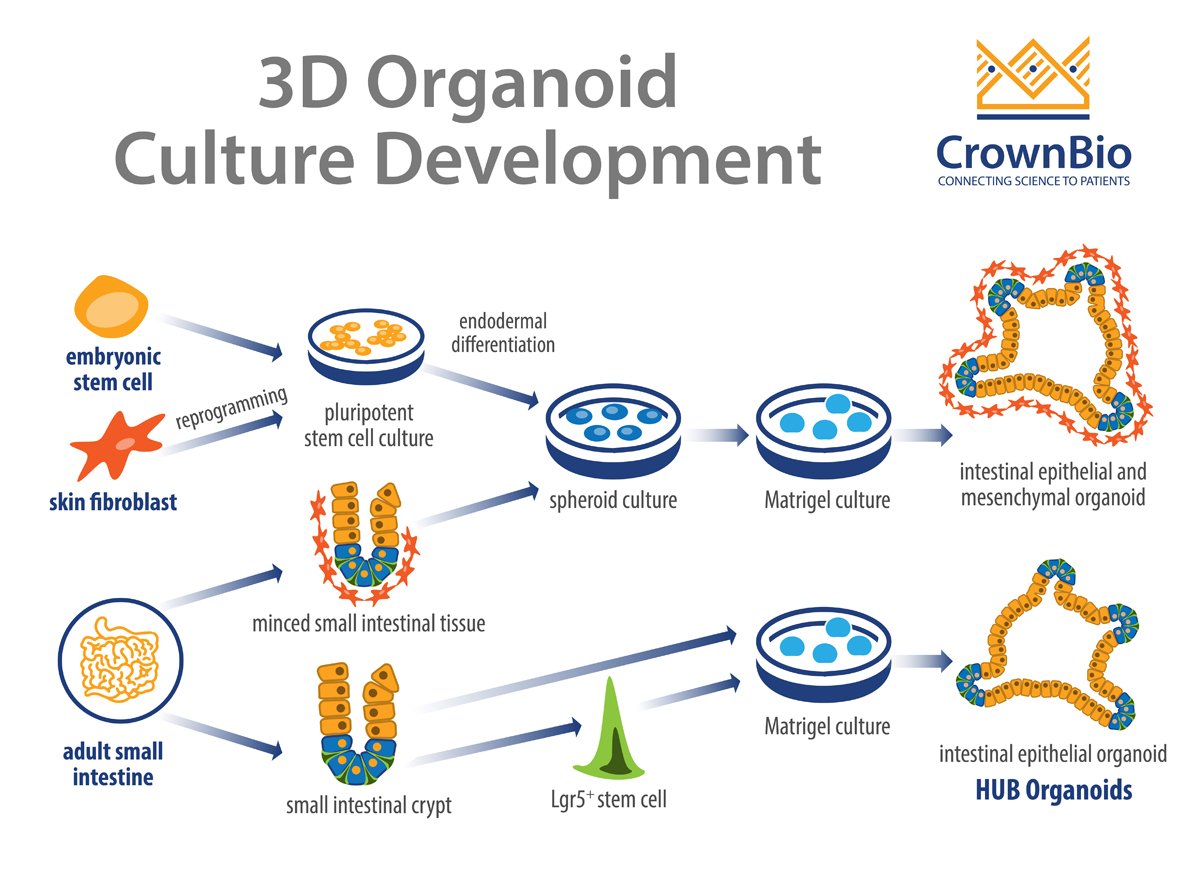This detailed illustration by Crown Bio, titled "3D Organoid Culture Development," showcases the comprehensive process of developing organoid cultures. Crown Bio's logo, a blend of a DNA strand and a crown, along with their motto, "Connecting Science to Patients," is prominently displayed in the top right corner. 

The diagram meticulously explains each step starting from various sources, including Embryonic Stem Cells and Skin Fibroblasts, which are reprogrammed into Pluripotent Stem Cell Culture. This progresses through several stages: Endodermal Differentiation, Spheroid Culture, and Matrigel Culture, ultimately resulting in an Intestinal Epithelial and Mesenchymal Organoid.

Additionally, the process includes starting material from the adult small intestine, which undergoes mincing to extract small intestinal tissue. From there, it isolates Small Intestinal Crypt, identifying LGR5 Stem Cells that are cultured to form Intestinal Epithelial Organoids. The bottom section of the illustration highlights these two pathways, emphasizing the creation of either Intestinal Epithelial and Mesenchymal Organoids or Intestinal Epithelial Hub Organoids. This visual flowchart effectively bridges the complex scientific procedures from initial cell sources to final organoid structures.